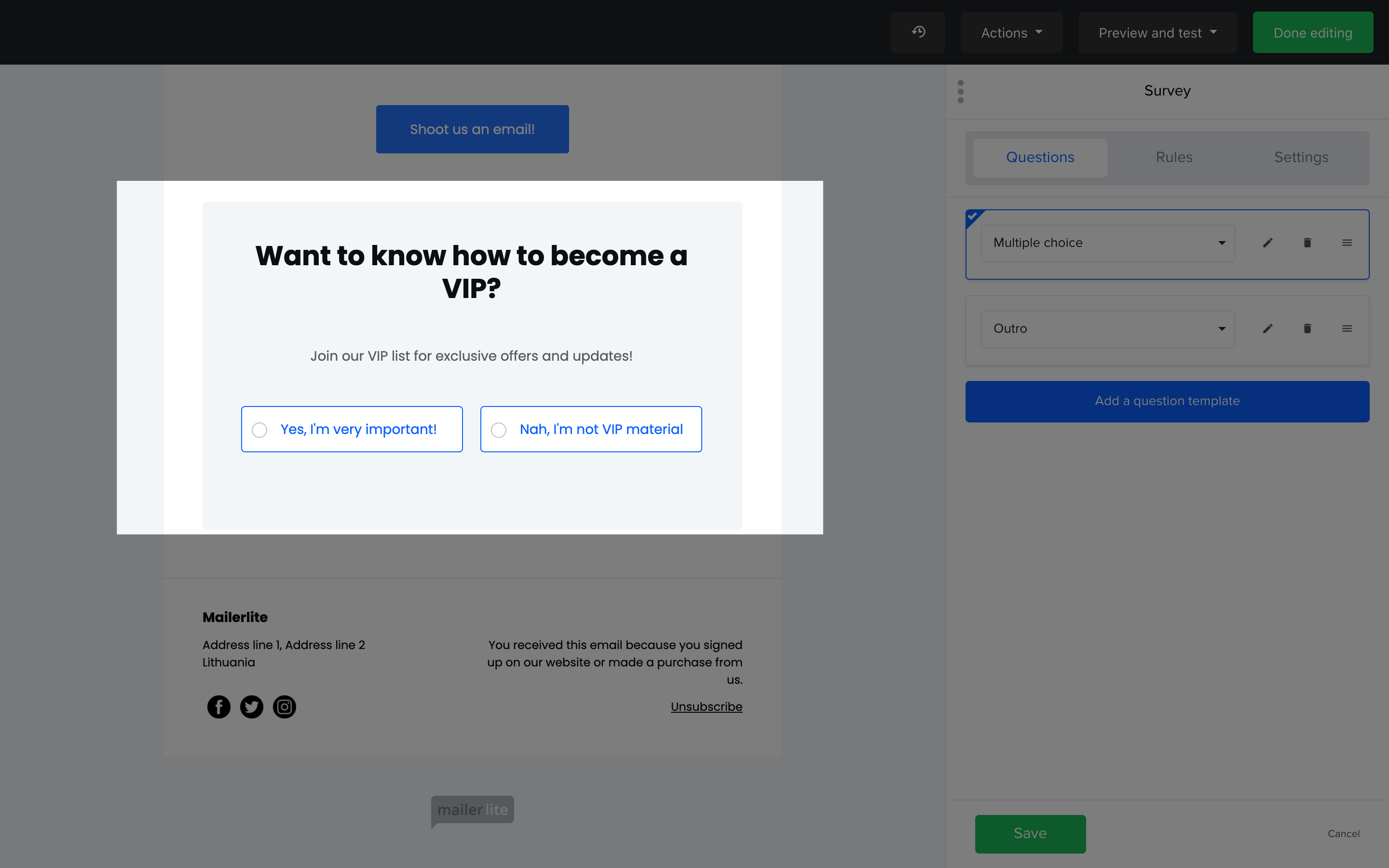The image showcases a main page with a pop-up menu on the right side. On the left side of the pop-up menu, there is a promotional message inviting users to join a VIP list for exclusive offers and updates. The message reads, "Want to know how to become a VIP? Join our VIP list for exclusive offers and updates." Below this message, there are two blue buttons: the left button says, "Yes, I'm very important," and the right button says, "No, I'm not VIP material."

The main background of the page has a light, generic header text that suggests an email or certain advice is needed. The pop-up menu's bottom left section includes fields for "Mailing address, Address line 1, Address line 2," and also features icons for Facebook, Twitter, and Instagram that are colored black.

On the right side of the pop-up, it states, "You received this image because you signed up on our website or made a purchase from us." Below this is a blue "Subscribe" button. Further down, there is another section that includes a text that reads, "Multiple choice add a question template," with another blue button labeled "Add a question template." At the bottom of this section, there are two buttons: a green "Save" button on the lower left and a "Cancel" button on the bottom right.

The header of the page features a black background with tabs on the top right including options like "Redo Action, Preview, Test, and Done Editing," with the "Done Editing" button highlighted in green.